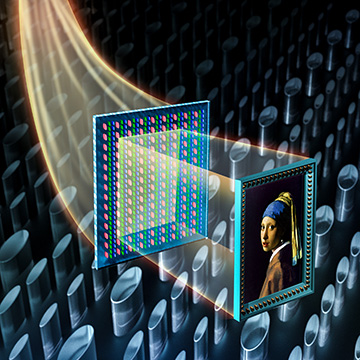The image is a highly detailed 3D graphic art piece. It features a central rectangular prism with golden-orange light beams penetrating it, which refract and scatter into smaller colored lights—specifically pink, green, and blue dots that are arranged in repetitive rows. Behind this prism, there is a blue picture frame adorned with gold tacks, containing a computerized drawing of a woman. The woman has her hair tied up in a ponytail and wears a large blue and yellow bandana across her forehead. She is dressed in a brown suit jacket over a white dress shirt, with red lipstick, and is turning her head to look directly at the viewer. Additionally, the background includes abstract elements resembling bent barrels with a metallic blue-silver hue, evoking the shape of old-fashioned typewriter keys. The overall composition includes another empty frame and visible laser-like light paths connecting the elements, adding complexity to the scene.